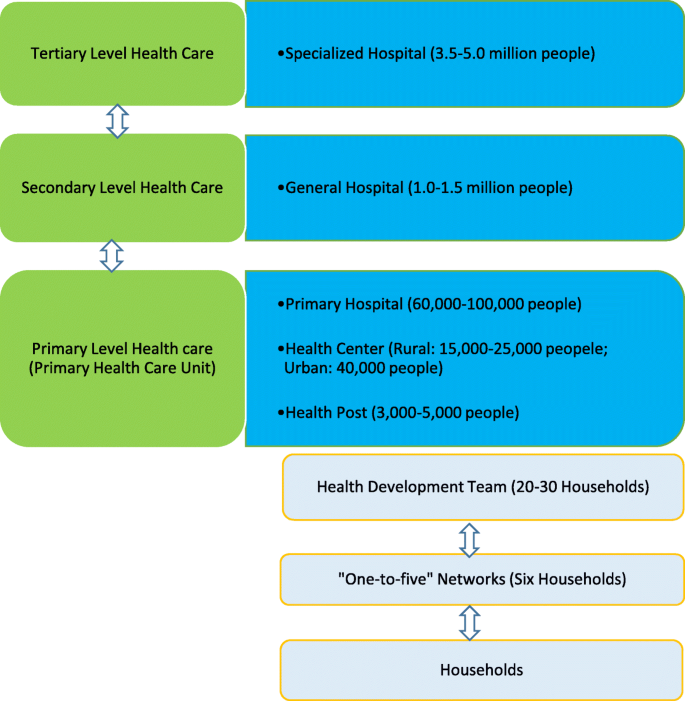The diagram illustrates the organizational structure of health care services, with distinct colored sections categorized by levels and corresponding population sizes. On the left-hand side, there are three vertically aligned green blocks labeled "Tertiary Level Health Care," "Secondary Level Health Care," and "Primary Level Health Care" (also referred to as "Primary Health Care Unit"), each connected by two-way arrows outlined in gray.

To the right of these green blocks, there is a corresponding set of longer blue blocks. The top blue block lists "Specialized Hospital (3.5 to 5.0 million people)" with a bullet point. Below it, the next blue block indicates "General Hospital (1.0 to 1.5 million people)" with another bullet point. The third blue block contains three bullet points: "Primary Hospital (60,000 to 100,000 people)," "Health Center - Rural (15,000 to 25,000 people), Urban (40,000 people)," and "Health Post (3,000 to 5,000 people)."

Below these, three light gray sections are listed, each connected by two-way arrows. The top gray section is labeled "Health Development Team (20 to 30 households)," followed by "1 to 5 Networks ('1 to 5') (6 households)," and lastly, "Households," representing the smallest unit. This detailed division signifies the hierarchy of health care services, organized by population coverage and type of health facility.